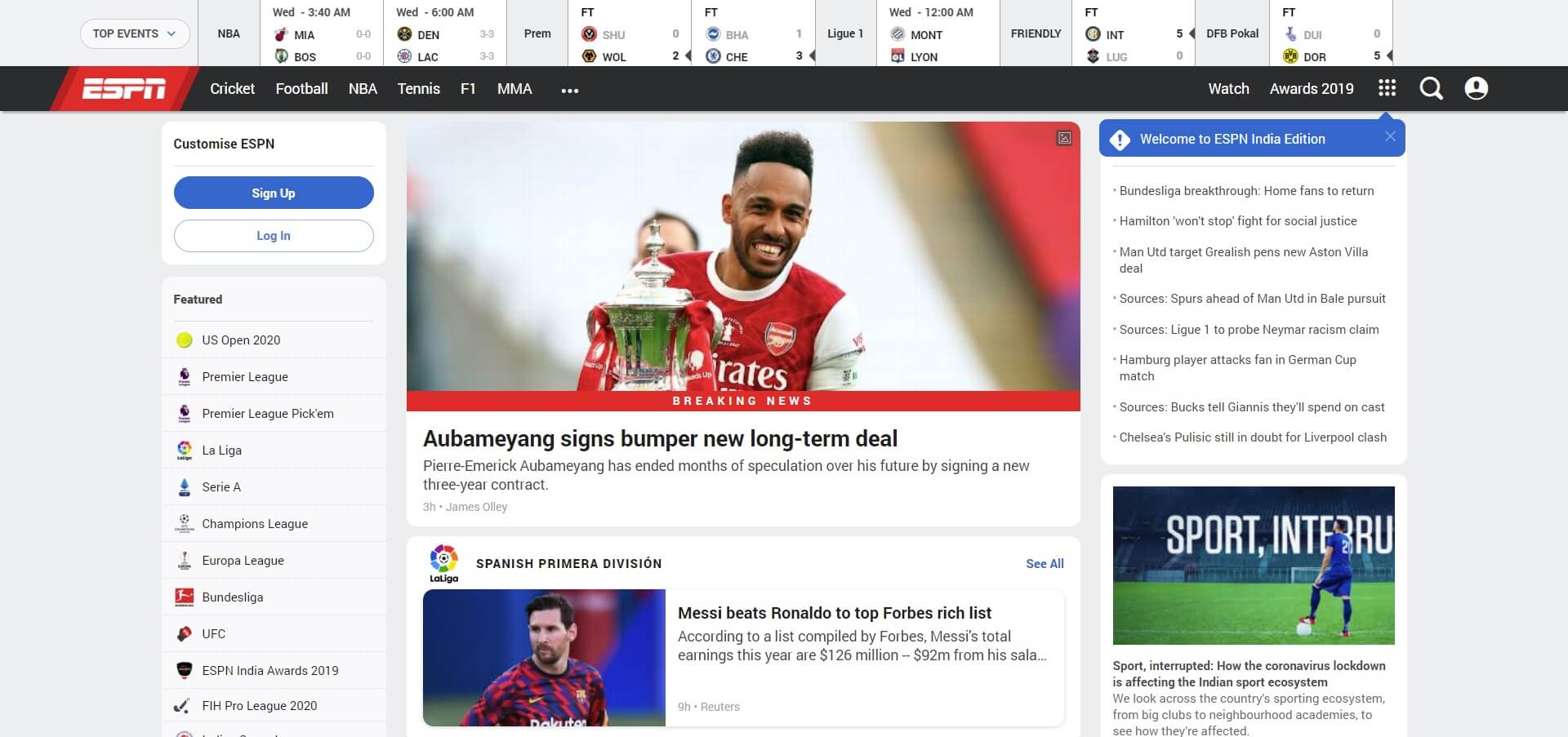This detailed image capture from the ESPN website features various sections, each presenting different sports scores, headlines, and news articles. At the very top, a navigation bar includes options such as "Top Events," "NBA," and displays current scores of ongoing NBA games. Below that, several additional sections display scores, though some text is unreadable.

One particular section titled "Friendly" is noted for showing scores, emphasizing its relevance to exhibition matches. Beneath a black separator line, another navigation bar lists various sports categories including "ESPN," "Cricket," "Football," "NBA," "Tennis," "F1," and "MMA." Further to the right on the navigation bar, there are links labeled "Watch" and "Awards 2019."

The body of the page contains several news articles with accompanying images. Notably, a picture of a soccer player holding a trophy, captioned "Aubameyang signs bumper new long-term deal," suggests contract news about the player Pierre-Emerick Aubameyang. Nearby, another image shows Lionel Messi, with a headline stating, "Messi beats Ronaldo to top Forbes Rich List," highlighting Messi's financial achievements over Cristiano Ronaldo.

On the right side of the page, a section labeled "Welcome to ESPN Inside Edition" features a blue background and several small-print headlines. Below this, there's a photograph of a soccer player standing on a field, with a partially visible backdrop featuring the text "Sport, Inter" which likely pertains to "Sport Interrupted."

The detailed elements reflect a dynamic and information-rich webpage catering to sports aficionados, providing instant updates, detailed articles, and various multimedia content all centralized on ESPN’s platform.